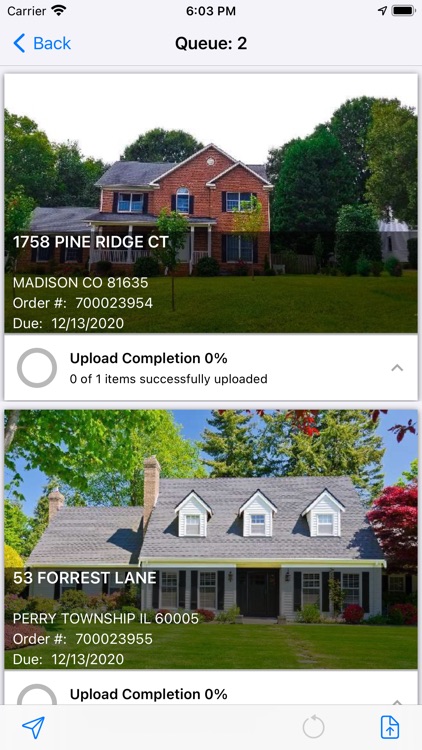The image is a screenshot from a mobile phone interface. In the top left corner, the status bar displays the cellular carrier name and signal strength. At the center top, it shows the time as 6:03 p.m. In the top right corner, there is a battery icon.

Below the status bar, there is a navigation header featuring a blue "Back" button with a back arrow underneath the time display. The text "Q2" is prominently positioned below this navigation header.

Underneath "Q2," there are two photographs accompanied by detailed information. The first photograph showcases a red brick, two-story house with a front porch, surrounded by trees and grass. The associated text reads: "1758 Pine Ridge Court, Madison, CO 81635, Order Number 700023954, Due 12-13-2020." Below this text, there is a progress bar labeled "Upload Completion" indicating zero percent, with the note "0 of 1 item successfully uploaded."

The second photograph depicts a white, two-story house also framed by grass and trees. The text for this entry states: "53 Forest Lane, Perry Township, Illinois 60005, Order Number 700023955, Due 12-13-2020." Similarly, this entry has an "Upload Completion" bar showing zero percent completion.

At the bottom of the screen, two buttons are visible: a "Send Mail" button located in the bottom left corner and an "Upload Document" button situated in the bottom right corner.